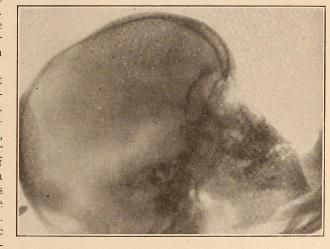This is a black-and-white, or grayscale, photograph, approximately two inches by two inches, framed by a thin, tan border. The image, which may have come from a medical journal or newspaper, has yellowed with age. At the center is what appears to be an X-ray or scan of a human skull, captured from a tilted angle, suggesting that the person was leaning back with their head propped upwards, facing slightly to the top right. The background of the image is empty, with no additional objects, text, dates, or labels present. Dark lines within the image suggest that it could also potentially be a drawing or an artistic rendering. Overall, the scan of the skull is very detailed, showing the bones clearly, and is the sole focus of this small, aged photograph.